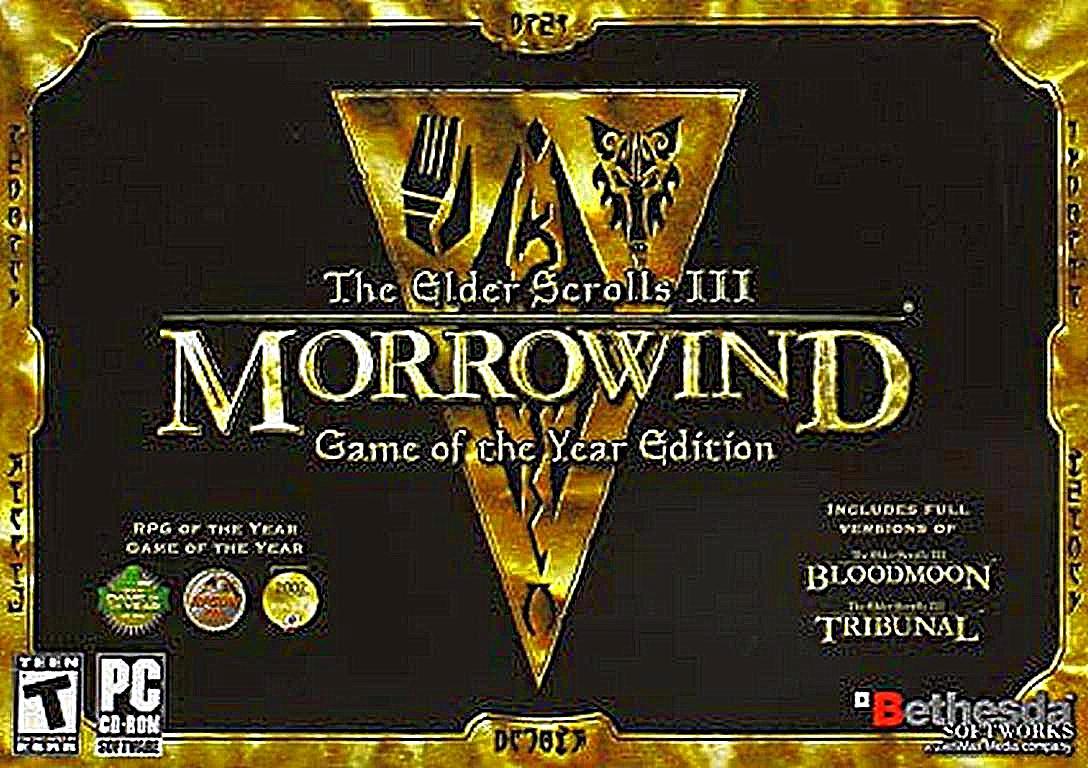The image is an advertisement for a video game characterized by a gold-colored, shining border. The central background is predominantly black and features an upside-down triangle adorned with various sketched items, including a bent fork-like shape on the left and an owl-like figure on the right. Superimposed on the triangle is the text "The Elder Scrolls III," followed by a bold line and large font reading "Morrowind," with the "M" and "d" more prominent, and beneath that, "Game of the Year Edition." The lower left corner displays a white square with a "T," signifying "Teen," and adjacent to it, another square indicating "PC CD-ROM" software. Above this section, small, pixelated text reads "RPG of the Year" and "Game of the Year," flanked by three circles in green, orange, and yellow, the text within them too blurred to decipher. On the bottom right, it states "Bethesda Softworks," with the text immediately above it mentioning that the package "includes full versions of Blood Moon and Tribunal." The overall image quality is extremely degraded, with much of the text being pixelated and difficult to read.